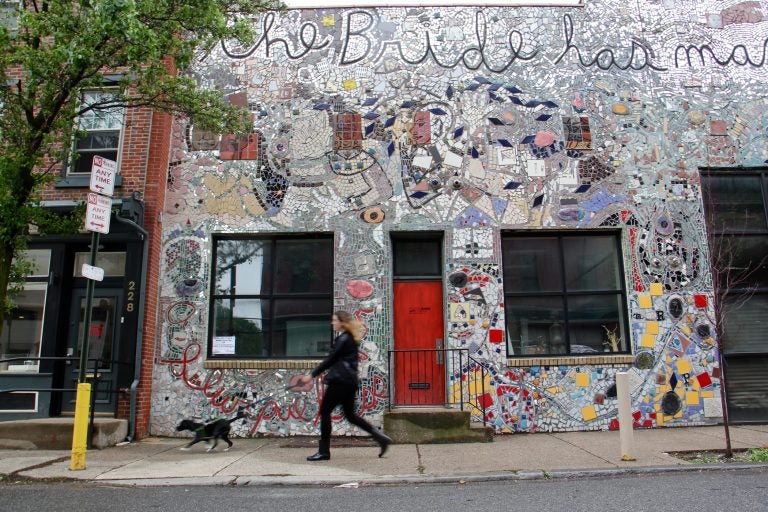This outdoor scene captures a vibrant, artistic street setting. In the foreground, a young woman dressed in black from head to toe, including a jacket, pants, and boots, is seen walking a small, energetic black dog on a leash along the sidewalk. Her long blonde hair flows as she walks, with her dog eagerly pulling ahead of her. Directly behind them is a distinctive building adorned with colorful and abstract wall art. The building's cement walls showcase an array of colored tiles forming artistic pieces, featuring faces, shapes, and patterns in shades of gray, black, red, yellow, blue, and white. This building also has two square windows and a bright red door, above which partially visible black lettering reads "the bride has". A no parking sign is positioned in front of the dog, adding to the urban vibe. To the left, there's another building with a red-brick facade and a large black metal door, marked with the number 228. This scene, vibrant with artistic expression and street life, suggests a hip, artsy neighborhood.